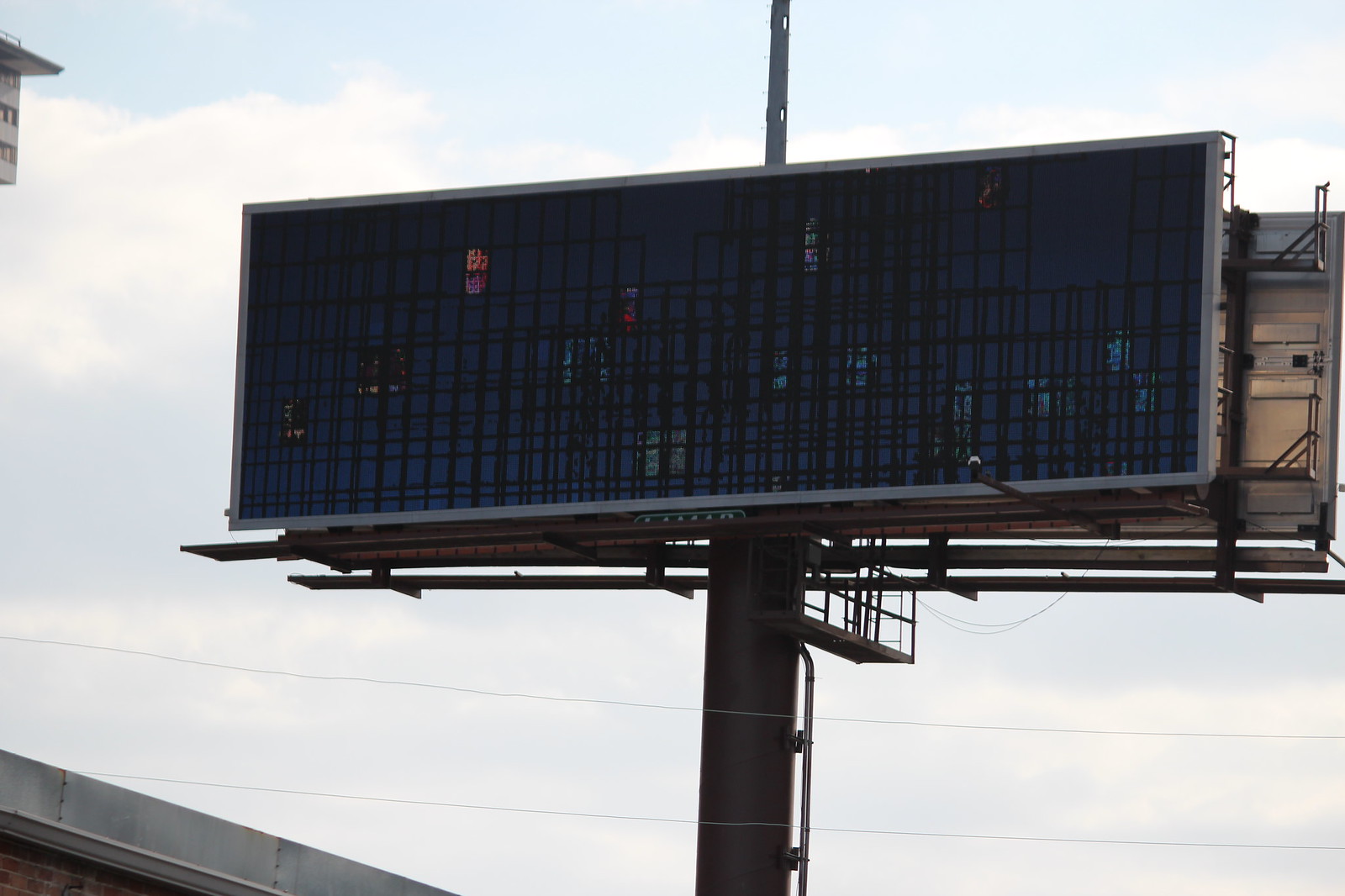This photograph captures a close-up view of a rectangular, billboard-style construction announcement board, mounted on a dark iron pole. The board itself is empty and black, overlaid with a wire mesh that features various colored Asian symbols resembling Chinese letters in vibrant shades of blue, purple, orange, red, and green. Visible in the image are two horizontal power lines running across the bottom of the board. The backdrop is a hazy, cloudy sky with patches of light blue, imparting a dull, overcast ambiance. In the corners of the image, the edges of a stadium with a cement and red brick structure, along with a rusty-colored back of another billboard facing the opposite direction, can be seen.